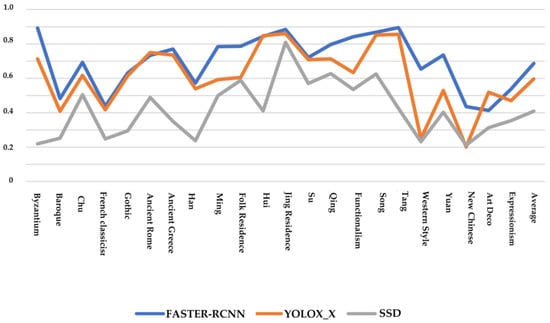This rectangular image features a detailed line graph with three distinct lines representing different data sets. The graph is plotted on a white, transparent background and is labelled along the vertical Y-axis with numerical values ranging from 0 to 1 in increments of 0.2. The horizontal X-axis is annotated with various historical periods such as Expressionism, Art Deco, and Ming and Han. The lines on the graph include: a blue line representing Faster R-CNN, a red/orange line signifying YOLOX-X, and a gray/silver line for SSD. Each line fluctuates in accordance with the labeled historical periods on the X-axis, creating a dynamic visual of how these data points vary over time. Both axes feature clear labels, although the descriptions at the bottom of the graph are small and vertically placed, making them hard to read.